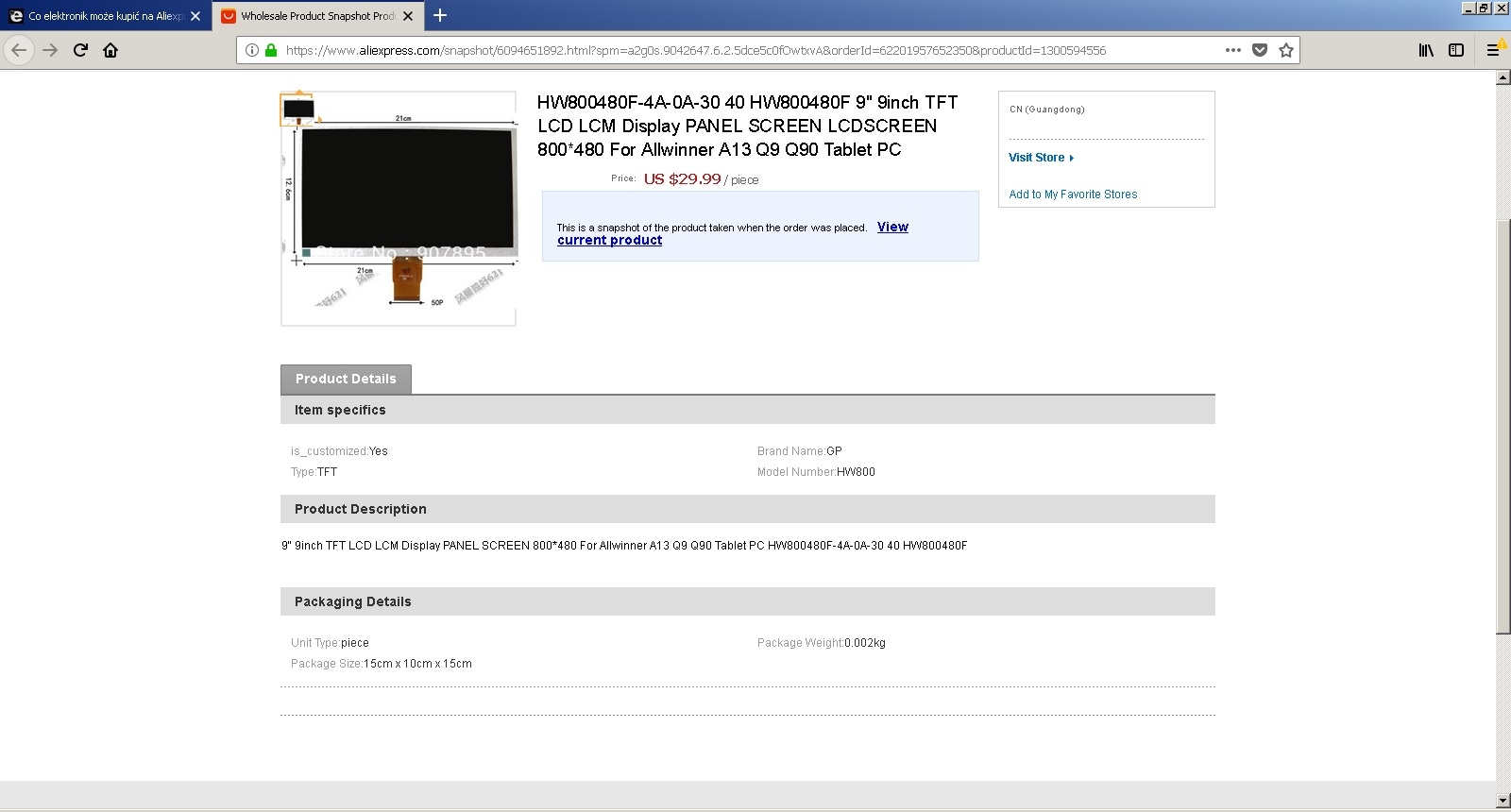A screenshot of a website displayed in landscape mode on a likely monitor or laptop screen is shown. The web page has a clean white background with a top border that features a gradient transitioning from dark blue on the left to light blue on the right. At the far left of this border, there's a small Internet Explorer icon, suggesting the browser used.

In the upper right corner, three indistinguishable buttons, presumably for shrinking, enlarging, and closing the window, are visible but too small to confirm. Below the border, a gray tab is open, displaying partial text likely related to wholesale. Beneath this tab, a gray bar stretches across the screen, featuring back, forward, refresh, and home icons on the left, along with a long white search bar that includes a security padlock icon and a lengthy URL, indicating the page could be secure.

The content of the web page appears to be from an e-commerce site specializing in electronics. It prominently displays a detailed diagram of a monitor or display screen characterized by a black rectangle representing the screen and a wood-tone brown stand. Dimensions are indicated with lines and arrows. The product model, labeled as "HB00480F," has a full descriptor reading "9-inch TFT LCD LCM display panel screen LCD screen for tablet PC," priced at $29.99 USD.

Below, a blue box contains further product details and blue underlined links, likely providing additional information such as "View Current Product." Scanning further down, sections labeled "Product Details" and other headings are visible but too small to read clearly, including terms like "Product Description" and "Packaging Details."